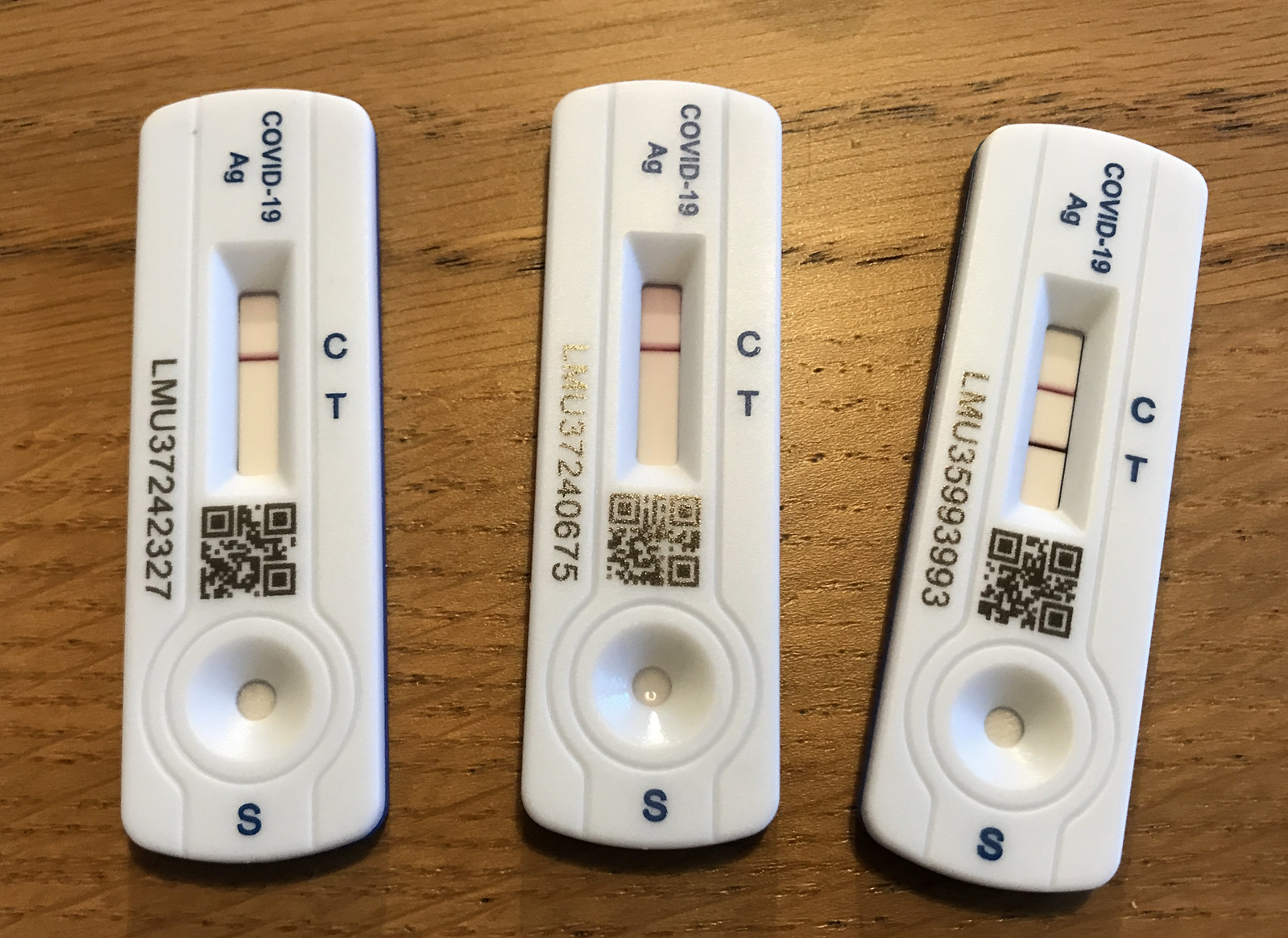This photograph showcases three COVID-19 antigen tests positioned vertically on a light oak wooden table. The tests, labeled "COVID-19 AG" in black lettering at the top, each present a different result. 

- **Left Test:** Displays a single red line at the 'C' (control) mark, indicating a negative result.
- **Middle Test:** Also shows a red line at the 'C' mark, confirming another negative result.
- **Right Test:** Features two lines, a red one at the 'C' mark and a black one at the 'T' (test) mark, indicating a positive result. This test is slightly askew, pointing towards the right.

Each test includes black metallic-looking QR codes, with the QR code on the middle test appearing golden in hue. Below the test window, the ID number "LMU 37242327" is printed. At the bottom of each test, there is a small indent for the liquid sample, marked with a black 'S'. 

The exacting detail of the test components, right down to the slight variations in the metallic finish of the QR codes and the colors of the lines, captures the nuances of these diagnostic devices laid out on the textured surface of the wooden table.